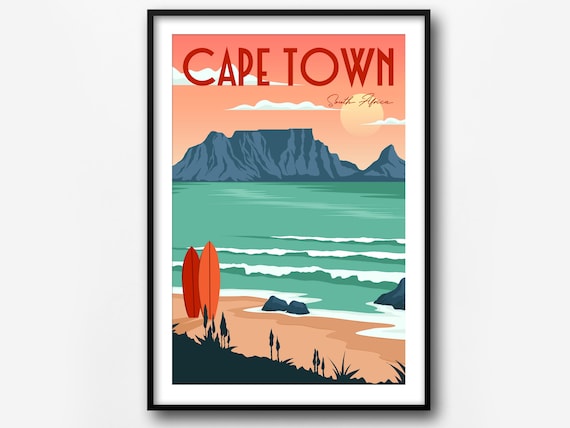The image is a color photograph of a framed portrait print hanging on a white wall. The print is encased in a narrow black frame with a wide white matting. The artwork inside, likely a lithograph, features a vivid beach scene and prominently displays "Cape Town" in large red letters at the top, followed by "South Africa" in smaller script below. The background of the image is a pinkish sky with wispy white clouds and a large orange sun. A gray, rocky mountain extends from the left to the right, its silhouette flat on the top with occasional pointed peaks. A green body of water, resembling the sea, sends crashing waves onto the sandy shore in the foreground. The beach features two surfboards, one red and the other orange, planted upright in the sand on the left side. Additionally, there are rocks scattered on the right and a patch of black brush with little weeds in the lower left corner. The overall impression of the scene is both serene and dynamic, capturing the essence of Cape Town's coastal beauty.